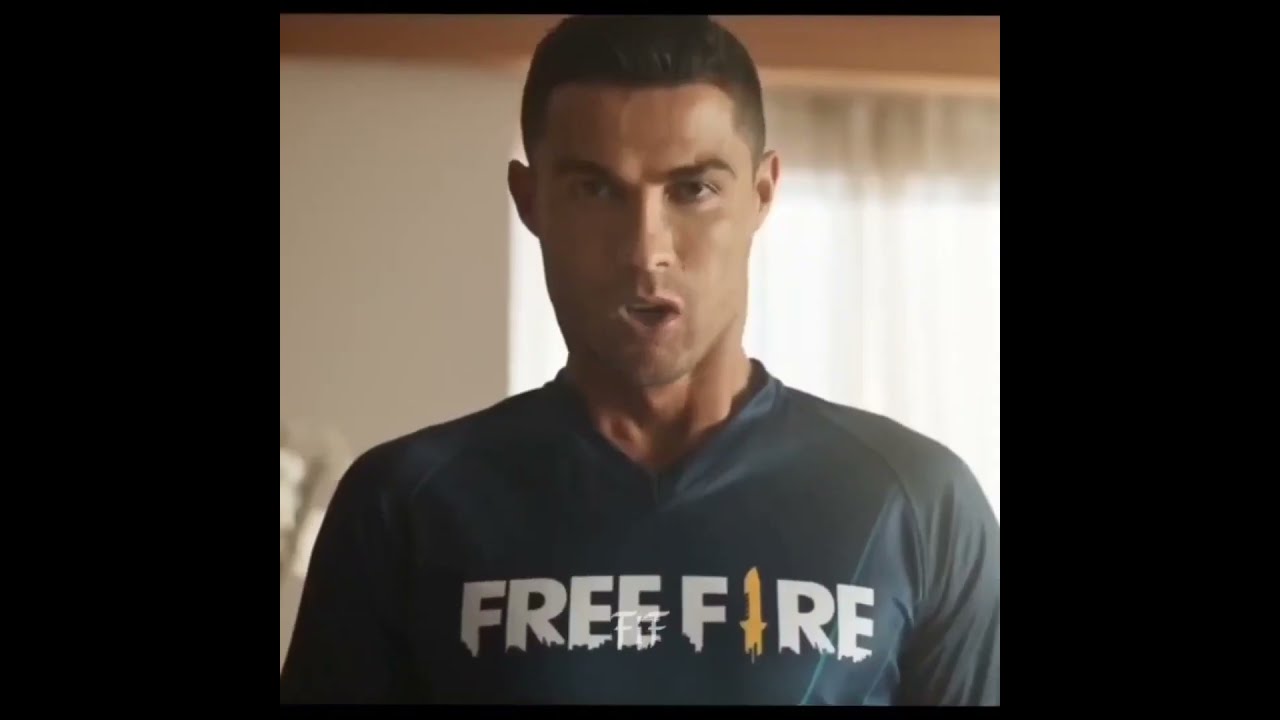A man stands directly in front of a window, framed in a square shot, as if captured from a YouTube video or advertisement. He appears to be either white or light-skinned, with short brown hair and no beard, giving him a clean-shaven, military-esque buzz cut. His facial expression shows determination and slight anger, with furrowed eyebrows and his mouth open mid-speech, forming a triangular shape. He is wearing a grey T-shirt with long sleeves that features the words "Free Fire" printed across the chest in white block letters, except for the letter "I," which is uniquely represented as a yellow or gold, skinny vertical rectangle or knife-like icon. The letters on the T-shirt are slightly frayed at the bottom. The background is unembellished with a white wall to his left and a window with a translucent white curtain to his right, emitting a bright light from outside, contributing to a rather bland and simple setting.